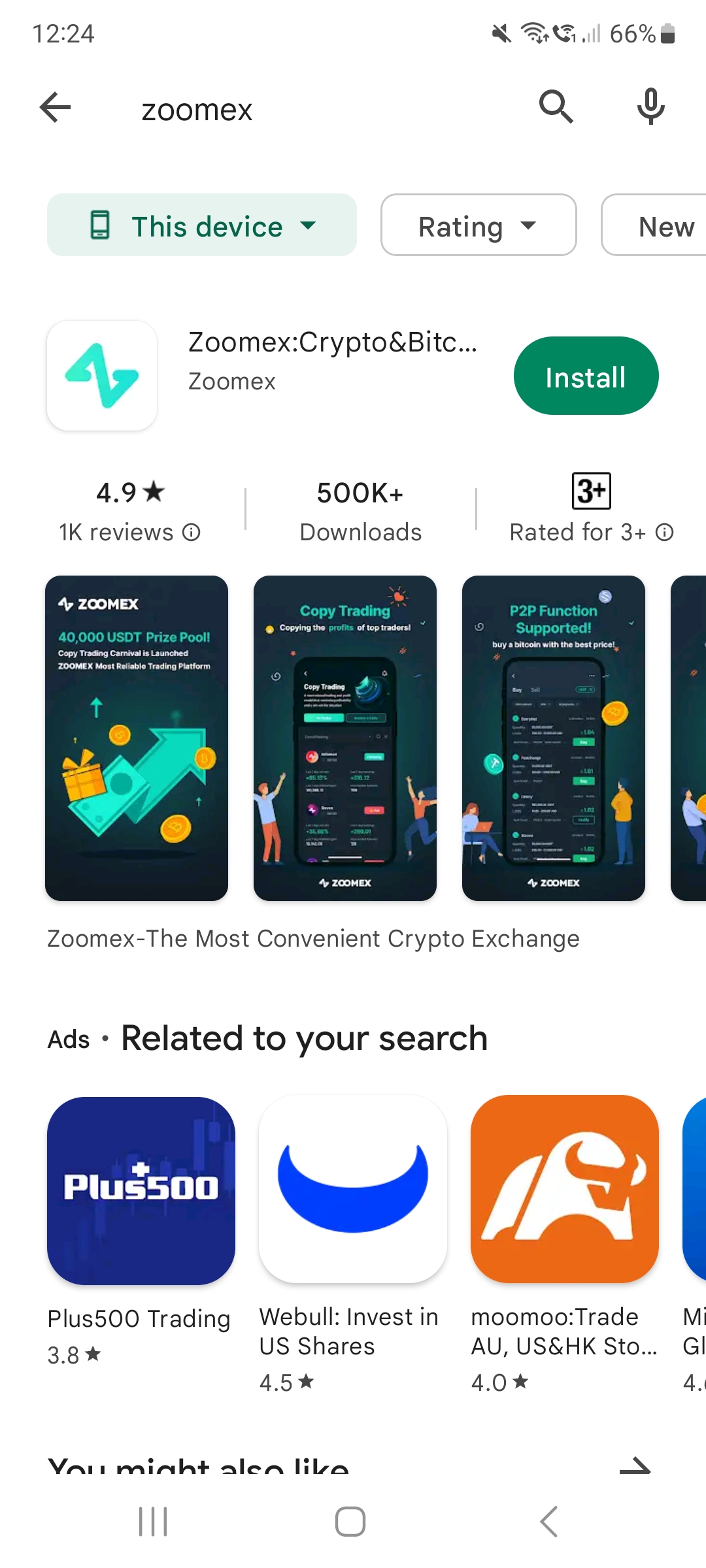This is a detailed screenshot from an app store, likely the Google Play Store or Apple App Store. In the search bar at the top, the text "ZoomX" (spelled Z-O-O-M-X) is entered. The displayed result is for the "ZoomX - Crypto and Bitcoin App," which is already installed on this device. The app has received a high rating of 4.9 stars from 1,000 reviews and has over 500,000 downloads. It is suitable for users aged 3 and up. ZoomX promotes itself as the most convenient crypto exchange, and the screenshot showcases various app features through a series of in-app screenshots and graphic designs. Below this, there is a section titled "Ads related to your search," listing other relevant apps. These include "Plus500 Trading" with 3.8 stars, "Webull - Invest in US Shares" with 4.5 stars, and "Moomoo - Trade AU, US, and HK Stocks" with a 4.0-star rating. This organized layout makes it easy for users to find and assess related apps quickly.